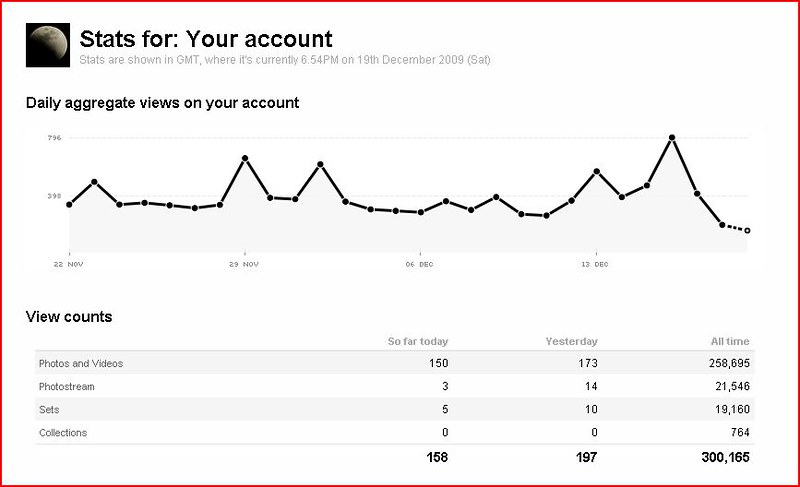The image is a detailed screenshot of a stats module from a dashboard with a red border. It features a white background and displays various metrics for an account. At the top left, there's a small avatar resembling a half-moon icon. The main headline reads "Stats for your account," followed by a gray subtext stating, "Stats are shown in GMT where it's currently 6:54 PM on 19th December 2009, Saturday." Below this, a subheading reads "Daily aggregate views on your account," accompanying a line chart that fluctuates and spans dates from the 22nd of November to the 13th of December. Under this graph, a table presents view counts categorized by "Photos and Videos," "Photo Stream," "Sets," and "Collections." These categories are further detailed in columns labeled "So far today," "Yesterday," and "All time," showing respective numerical data such as photos and videos with counts like 150, 173, and 258,695 respectively.